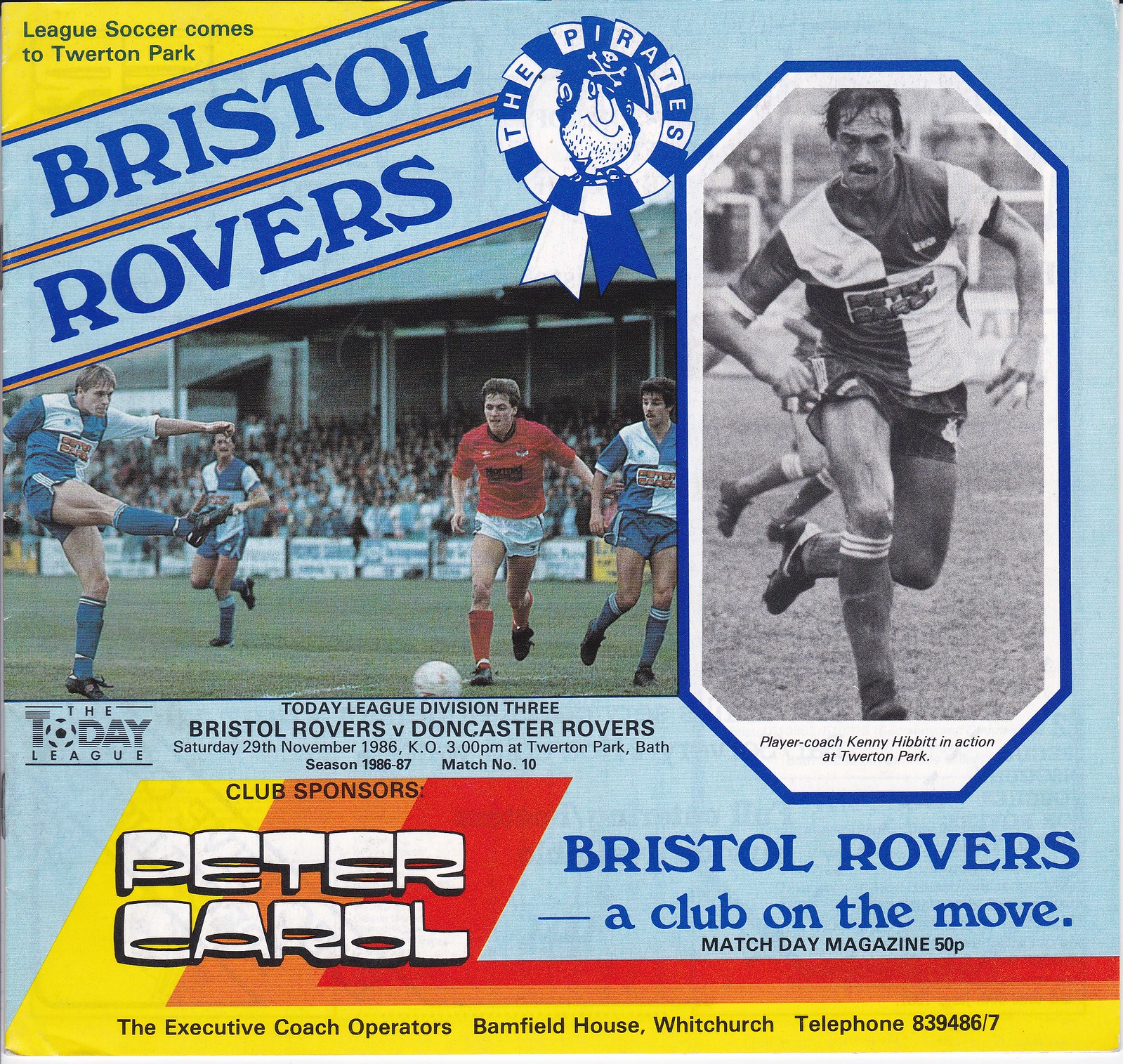The front cover of a Match Day magazine for the Bristol Rovers is vibrant and colorful, featuring a light blue background accented with yellow, orange, and red stripes. Dominating the upper left corner is the headline "Lee Sokka comes to Thwaiting Park." Below it, the title "Bristol Rovers" is prominently displayed, followed by a circular ribbon graphic featuring an illustration of a pirate, captioned "The Pirates." Adjacent to this ribbon, there's a black and white photograph of a soccer player running, identified as Player Coach Kenny Hibbert, with the caption indicating his action at Thwaiting Park. Another key visual on the cover is a dynamic, colored image of a soccer match showing players from two different teams – one in blue and white jerseys and the other in red jerseys with white shorts. The ball is actively in play, with spectators visible in the background. Information about the match between Bristol Rovers and Doncaster Rovers, the sponsorship details, and the price of the magazine (50p) are also featured, all contributing to the vibrant and information-rich design of the magazine cover.